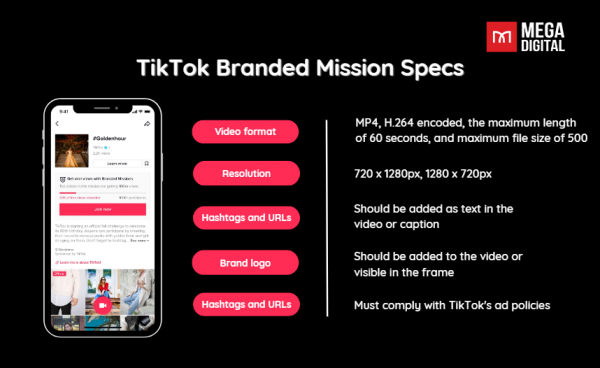The image features a prominent red square that displays the text "Mega Digital" in white. Adjacent to it, the words "TikTok Brand Admission Specs" are clearly visible. On the left side of the image, there is an illustration of a gold-colored smartphone with directional arrows indicating left and right, along with various text labels such as "address", "stairs", and more black text.

Further details include a red rectangle that prominently states "Join Now" and another section that encourages viewers to "Learn More About TikTok." Scattered throughout the image are pictures of people either standing or sitting on various objects.

Additionally, a red circle containing a white square resembling a camera icon is present. There are also several ovals with text; one says "Video Format," another "Resolution," and a third "Hashtags and URLs." 

The specs within the image provide specific guidelines for TikTok brand videos:
- Video format must be in MP4, encoded with H.264.
- Maximum video length is 66 seconds.
- Maximum file size allowed is 500MB.
- Resolutions specified are 720x1080px and 2080x720px.
- Text including hashtags and URLs should be added to the video caption or be visible within the frame of the video.
- All content must comply with TikTok's ad policies.